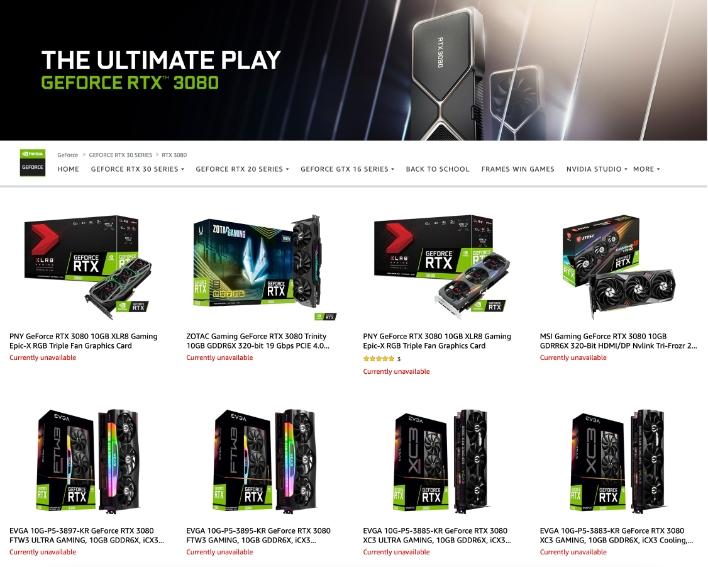The top part of the image features a visually striking banner. On the mid-right section, the banner showcases a gaming pack, identifiable by geometric black shapes transitioning from triangles into squares. These shapes are overlaid with white text. Backing this display is either a second similar image or a reflection.

The banner is traversed by white lines and begins with a black background on the left side, gradually transitioning into a brightly illuminated look towards the top right, simulating light emanation. Prominently in the center of the banner, large white capital letters in a digital font proclaim "THE ULTIMATE PLAY". Directly beneath this, in the same digital font but in a vibrant lime green, it reads "GEFORCE RTX 3080".

Beneath the banner, the website has a white background and features a horizontal menu bar. The menu items, written in black capitalized fonts, start with "HOME" on the far left and continue with "GEFORCE RTX 30 SERIES" which includes a drop-down arrow, followed by "GEFORCE RTX 20 SERIES" also with a drop-down arrow, "GEFORCE GTX 16 SERIES" with another drop-down arrow, then "BACK-TO-SCHOOL", "FRAMES WIN GAMES", "NVIDIA STUDIO" with a drop-down icon, and a section marked "MORE" that also includes a drop-down icon.

Below the menu, there are eight different product images. The first product is titled "PNY GeForce RTX 3080 10GB XLR8 Gaming EPIC-X RGB Triple Fan Graphics Card".